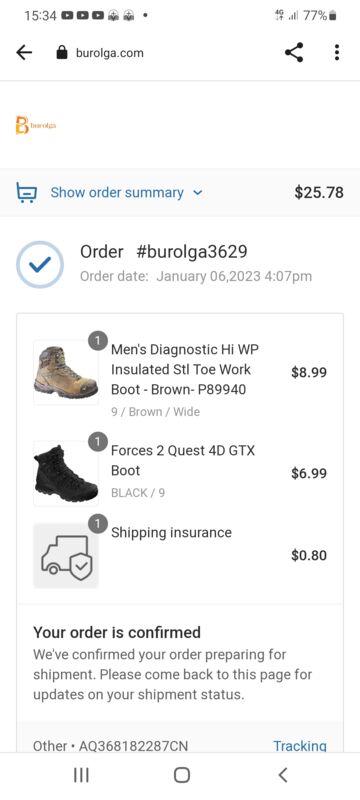A man is ordering an item from his smartphone using a website displayed in military time, specifically 15:34. The screen captures various details of the order process. At the top of the display, several icons are visible, one of which resembles YouTube, alongside two other unrecognized circular icons. Additional indicators suggest the user is connected via a 4G network, has a 77% battery level, and has good signal strength.

The website address appears to start with "burl," possibly referring to "burlaga.com," although the exact URL is uncertain. The website is secured, as indicated by a padlock icon next to the address.

The order summary shows a total amount of $25.78 for an item labeled "Men's Diagnostic Age High Way P. Work Boot" in brown, priced at $8.99. Shipping and insurance cost $0.80, which suggests this is a partial order detail, potentially comprising only a single boot.

The order date is specified as January 6, 2023, at 16:07. The confirmation screen mentions that the order has been confirmed, and there is a "Tracking" option below, though no further tracking details are provided.